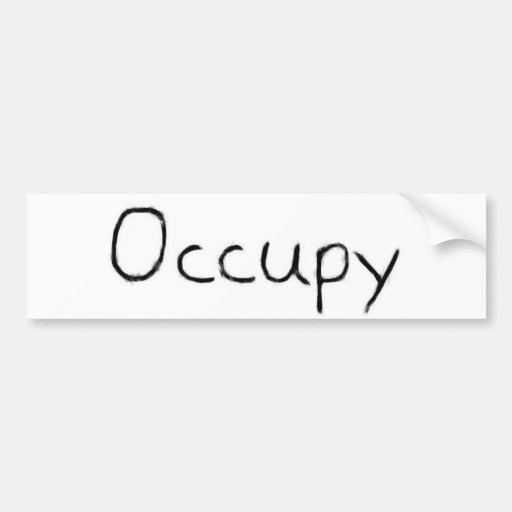The image showcases a small, nearly white, light grey background with a central bright white rectangular strip. This strip features the handwritten-style word "occupancy" in black letters, where the "O" is capitalized, and the rest are in lowercase. The black ink appears uneven, typical of a non-precise marker, with occasional spread. The top right corner of the white strip is curved, peeling away slightly, much like a sticker or a turning page, adding a tactile dimension to the flat surface. The strip's handwritten text, though computer-generated, captures an imperfect, personalized touch, with distinctive features like the two identical 'C's and the imperfectly circular 'O'.